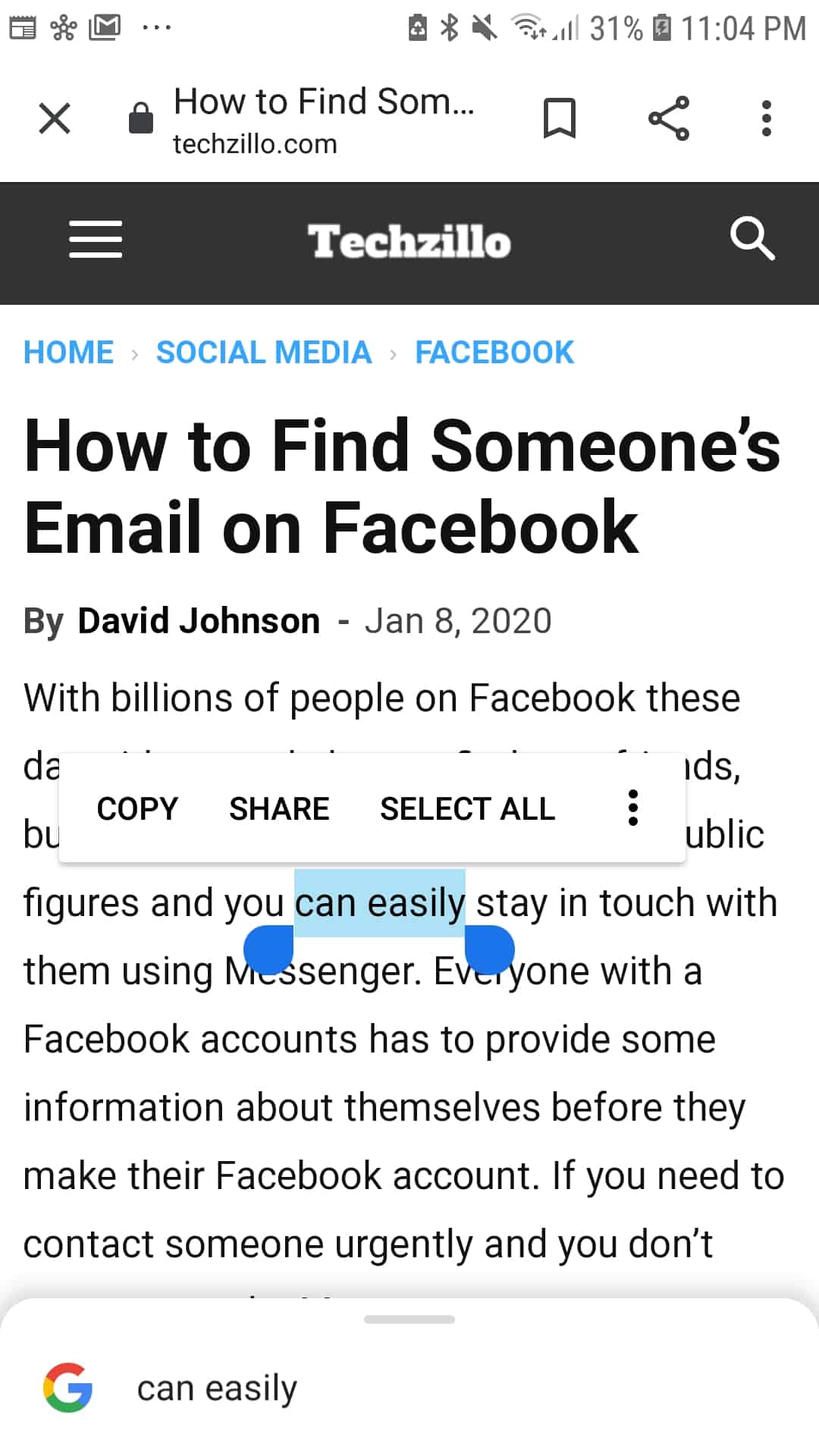The image appears to be a screenshot taken from a cell phone, displaying a webpage with a white background and black text. It primarily features a vertical, rectangular layout. At the top of the image, the address bar is visible, showing a partial query "how to find some SOM..." and the website "techzillow.com". Below this, there is a prominent black bar with the site's name "TechZillow" in the center and a magnifying glass icon on the right, indicating a search function.

The main content begins with a headline that reads, "How to Find Someone's Email on Facebook" by David Johnson, dated January 8th, 2020. This is followed by an introductory paragraph starting with "With billions of people on Facebook these..." before being partially obscured by a pop-up window. Skipping the lines obscured by the pop-up, the visible text continues with "figures and you can easily stay in touch with them using Messenger. Everyone with a Facebook account has to provide some information about themselves before they make their Facebook account. If you need to contact someone urgently and you don't..."

Additionally, certain text "can easily" within the article has been highlighted in blue. At the bottom of the screenshot, there is a Google bar featuring a small Google logo followed by the phrase "can easily," suggesting that someone might have been conducting a search or editing text.